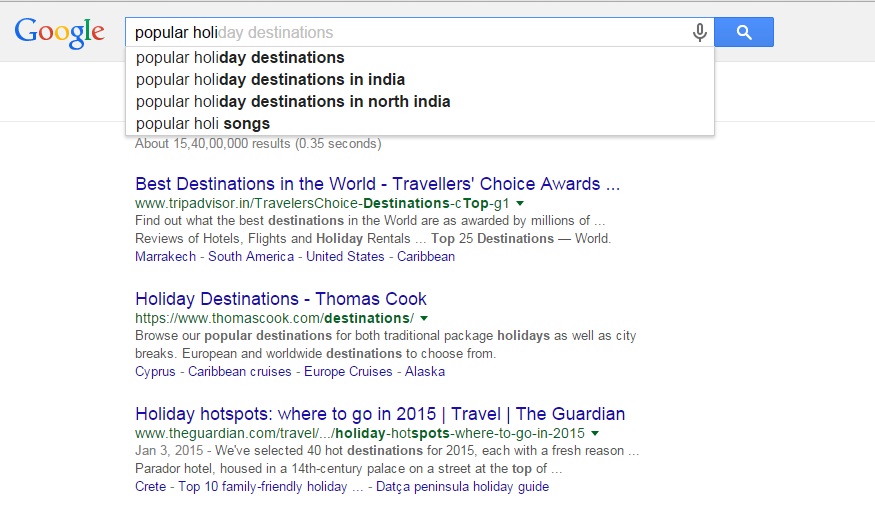This is a screenshot of a Google search page captured on a widescreen format, with a minimalistic white background that seamlessly blends into the browser's white screen. At the top of the page, a gray navigation bar is clearly visible, prominently featuring the Google logo on the left side in its iconic multicolored design. Within the search field, the user has entered "popular H-O-L-I," and Google’s autocomplete functionality suggests completing the phrase as "popular holiday destinations" in light gray text. 

Just below the search box, a list of related autofill suggestions appears, including options like "popular holiday destinations," "popular holiday destinations in India," "popular holiday destinations in North India," and "popular H-O-L-I songs."

Scrolling down, the search results are displayed, each present in the classic Google format. The first result is titled "Best Destinations in the World - Traveler's Choice Awards," linking to tripadvisor.in/india. The next entry is "Holiday Destinations - Thomas Cook" found at thomascook.com/destinations. The third result is "Holiday Hotspots: Where to Go in 2015 - Travel" from the British publication, The Guardian, suggesting this screenshot may date back to around 2015. Each result's title is in blue, the website link in green, and the description text in either black or gray, accompanied by blue hyperlinks for further information.